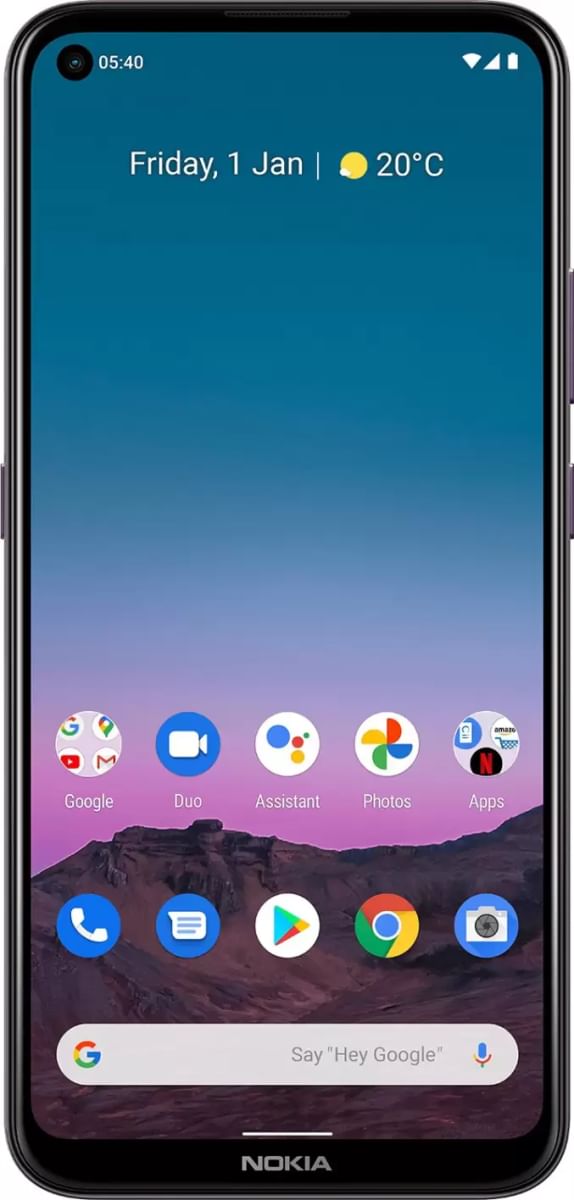The image depicts a Nokia cell phone displaying a screenshot. In the top left corner of the screen, the time is shown as 5:40. In the top right corner, three icons indicate signal strength, Wi-Fi strength, and battery life. The date is displayed at the top of the screen as "Friday, 1 January," followed by a separational line below which a sun icon indicates sunny weather with a temperature of 20 degrees Celsius.

Beneath this, the home screen contains two rows of app icons, with each row featuring five circular icons:
- Top row: Google, Duo, Google Assistant, Google Photos, and a folder containing the Netflix and Amazon apps.
- Bottom row: Phone, Messaging, Google Play, Chrome, and Camera.

Below the app icons, there is a Google search bar with a microphone icon for voice input, indicating that users can use voice commands by saying "Hey Google."

The Nokia phone has one button on the left side and two buttons on the right side.